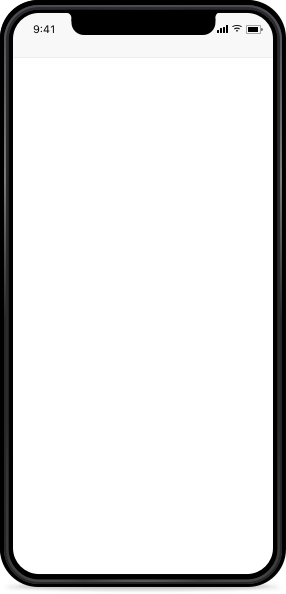This image is a photo of the front side of a black Apple iPhone. The screen is entirely blank, displaying a white background with the exception of a gray bar at the top. In the gray bar, the time is shown as 9:41 on the top left. The top right corner features several icons: a full-strength cellular signal icon, a full-strength Wi-Fi icon, and a battery icon indicating that the phone is almost fully charged but not currently connected to a charger. The phone itself is sleek with no visible edges, emphasizing a minimalist design.